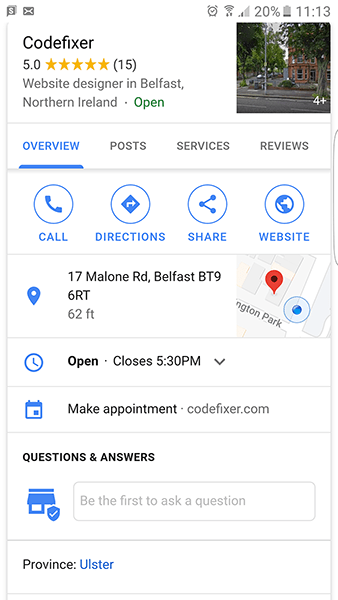This screenshot, taken from an iPhone, displays the search results for a business named "Code Fixer" in Northern Ireland. Code Fixer boasts an impressive five-star rating based on 15 customer reviews. The interface offers convenient buttons for making a call, getting driving directions, sharing the business details, or visiting their website directly. Further down, the screen provides essential information including the business address, a map view for easy navigation, the business hours, an appointment booking option, and a feature to submit inquiries.